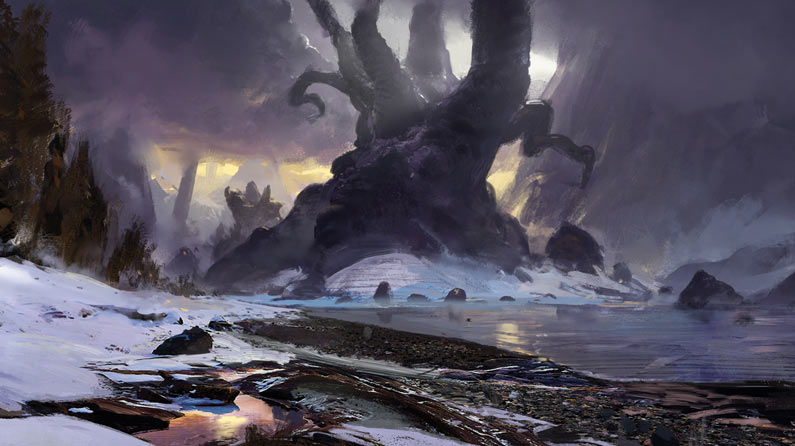The image presents a dark and surreal landscape that appears to blend photography with animation, creating a mythical atmosphere. In the foreground, there is a realistic depiction of a riverbank littered with dark brown detritus, logs, and muck, while patches of snow ascend the bank on the left side. To the right, a river with clouded water and a thin layer of fog meanders through the scene. Dominating the center is an enormous, gnarly tree, its thick, bare trunks extending upwards beyond the frame, standing on a snowy, icy island. The left side of the image is enveloped in thick, dark clouds with purples and dark greys, while behind the tree a thin strip of yellow light pierces through the murky skyline, topped by a whitish-grey obscured sky. The background features dark, mist-covered mountains with strange, almost tentacle-like shapes, and the overall color palette is dominated by bluey greys, contributing to the eerie, apocalyptic ambiance. The scene is devoid of any living creatures, enhancing the desolate, somber mood.